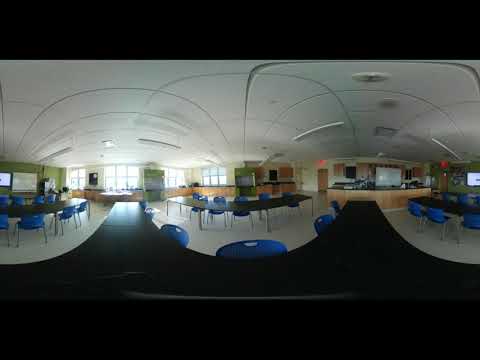The image depicts an interior space that appears to be a hybrid between a classroom, office meeting room, and a luncheon area. The room features several tables, approximately three, each accompanied by blue chairs, ranging from five to ten per table. Prominently, the space includes a larger, semicircular table also lined with blue chairs, facing what seems to be a screen setup for presentations or lectures. The environment is further characterized by green walls and blackboards or whiteboards situated on both sides. The floor is light white and the ceiling is similarly light-colored with built-in lights. Windows in the background allow natural sunlight to pour in, indicating a sunny day outside. Additionally, there is a decorative cutout in the foreground with three dips and two spikes, suggesting the viewer is peering through some kind of partition. The room appears empty of people at the moment, and an area resembling a lunch counter is visible in the right-hand foreground, reinforcing the multifunctional nature of the space as both an area for meetings and casual dining.